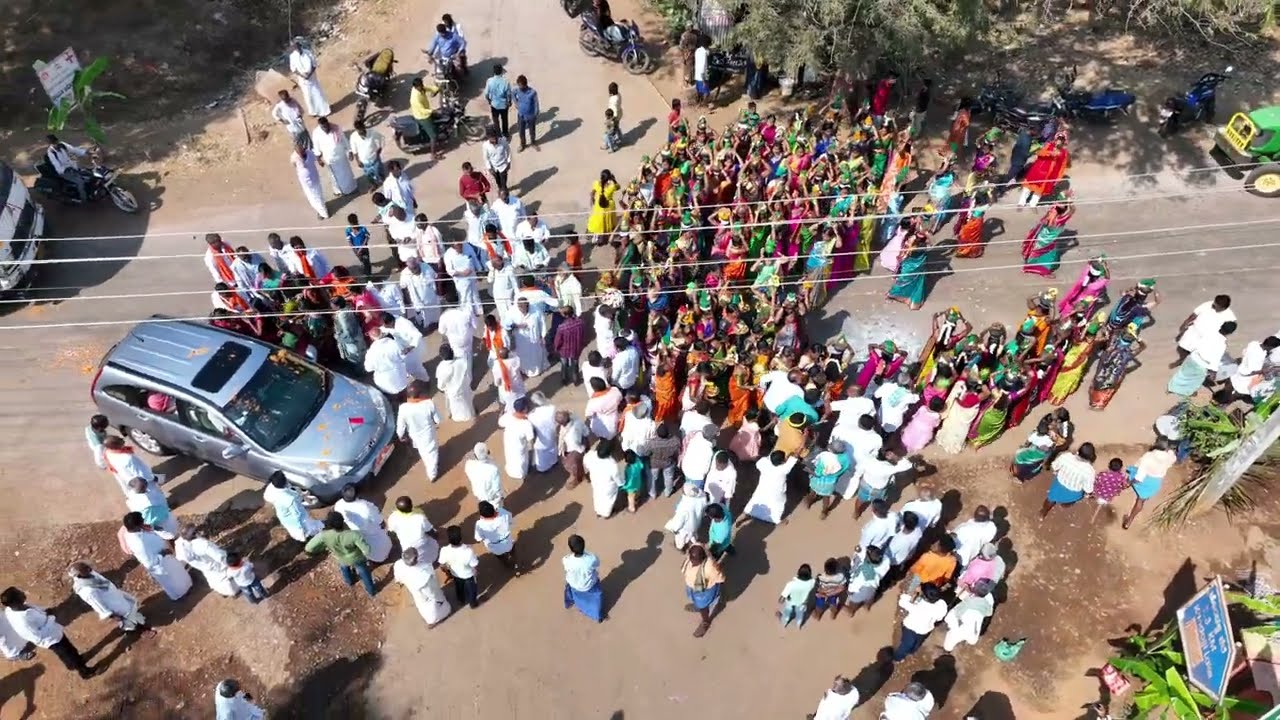The image is a vividly detailed, color photograph captured from a drone, providing an expansive overhead view of a bustling intersection in a foreign country, possibly India. The scene is dominated by a large group of people gathered in the middle of a paved, yet dusty road. The central focus is a silver van on the center-left side, which is being blocked by the crowd, presumably during a protest. The people are predominantly dressed in long, white robes, with some individuals in colorful, traditional Indian attire. Scattered motorcycles add to the congestion. 

The roadside is bordered by flat, padded-down earth, and tropical plants punctuate the otherwise dusty environment. Overhead, a network of telephone wires crisscrosses the intersection, adding to the scene's complexity. A small green tractor is partially visible in the top right corner, while a blue sign with indecipherable white text stands out in the bottom right. The photograph, an example of Photographic Representationalism and Realism, captures not only the physical chaos but also the charged atmosphere of the moment, highlighting the intersection between daily life and civil unrest.